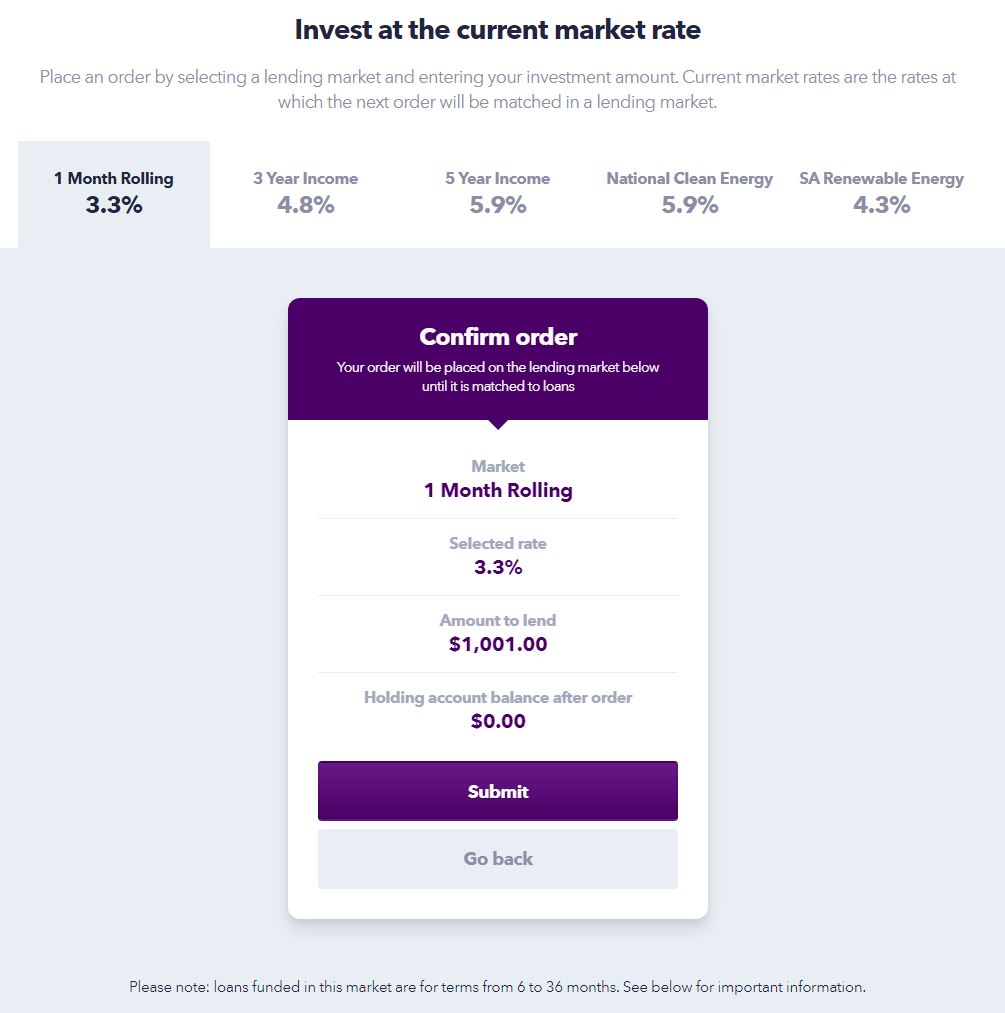This is a detailed screenshot of a financial app interface for investing in lending markets. At the top center of the screen, bold black text reads "Invest at the current market rate," with an instructional subtext in smaller black letters explaining, "Place an order by selecting a lending market and entering your investment amount. Current market rates are the rates at which the next order will be matched in the lending market."

Below this instructional text is a detailed chart with six tabs, each representing different investment options. The first tab, labeled "One Month Rolling at 3.3%," is currently selected. Under this tab is a small box with a purple header displaying "Confirm Order." It informs the user, "Your order will be placed on the lending market below until it is matched to loans." This section includes several rows with specific details:
1. Market: One Month Rolling
2. Selected Market Rate: 3.3%
3. Amount to Lend: $1,001
4. Holding Account Balance After Order: $0

Below these details, there is a purple "Submit" button and a grayed-out "Go Back" button, indicating the user can proceed with the order or return to the previous screen.

The other tabs at the top present different investment options with various returns:
- Three-Year Income at 4.8%
- Five-Year Income at 5.9%
- National Clean Energy at 5.9%
- SA Renewable Energy at 4.3%

At the bottom of the screen, outside the chart area, is a disclaimer in small letters: "Please note, loans funded in this market are for terms from six to 36 months. See below for important information."